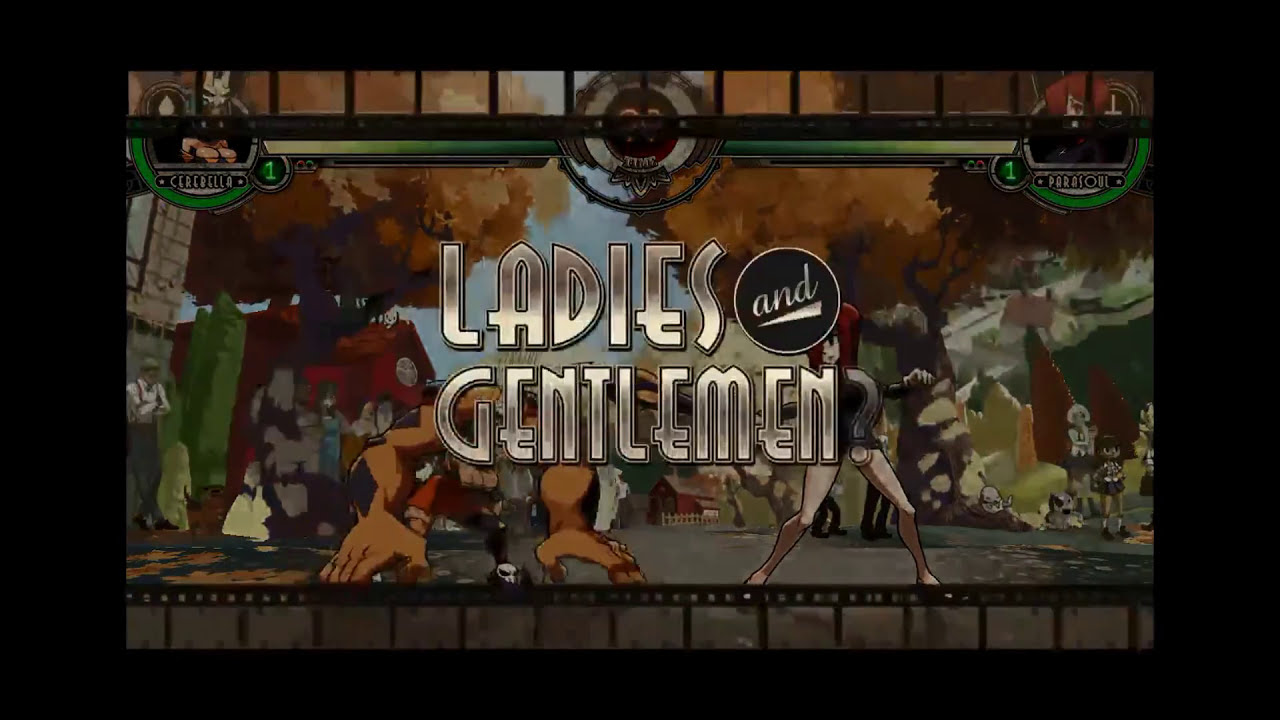This image is a detailed screenshot from a video game, featuring a stylized, anime-like scene framed by a black border. Dominating the center is the title "Ladies and Gentlemen" in a gleaming white, Art Deco-inspired font, with the word "AND" underlined and enclosed in a black circle with a silver ring. The backdrop depicts an autumn forest with orange-brown leaves. In front of this, on what appears to be a stage, stand two central characters: a tall woman with red hair in a black bodysuit and bare legs, positioned in a combative stance, and a brutish male figure with immensely large arms and hands, red shorts, and black triangle tattoos. They appear to be facing off. Flanking this main confrontation are various other figures: an adult gentleman in a suit and several young girls, watching the scene unfold. The top of the screen features a game-like interface with score indicators and character avatars, enhancing the impression that this is a captivating moment in an animated or video game experience.